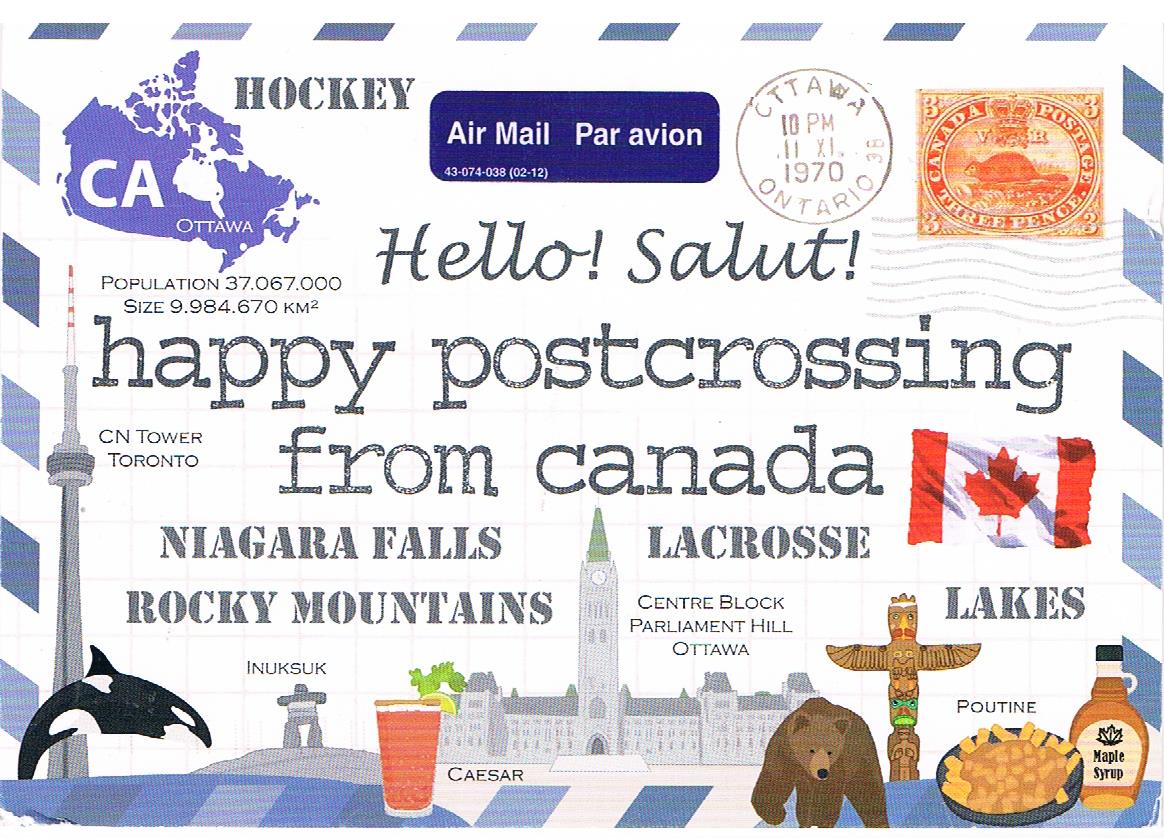This vibrant Canadian postcard features a lively blue and white candy cane stripe border. The top right corner boasts a reddish-orange Canadian postage stamp with a beaver motif, postmarked Ottawa, 10 p.m., 1970, Ontario. The top left corner includes the words "Hockey" alongside a blue map of Canada and the text "C.A. Ottawa." Centered prominently is "Air Mail Par Avion" and greetings in both English and French: "Hello, Salute, Happy Post Crossing from Canada."

The postcard is adorned with numerous Canadian-themed illustrations and landmarks. Notable mentions include the CN Tower in Toronto, Niagara Falls, the Rocky Mountains, the Centre Block on Parliament Hill in Ottawa, and various lakes. Cultural references are abundant, such as a drawing of an Inuksuk, a totem pole, a teepee, and traditional Canadian foods like poutine—with fries and cheese—and a bottle of maple syrup. 

Among the colorful depictions are a Canadian flag, a whale leaping from the water, a brown bear, a drink labeled as Caesar with a glass of red liquid and green garnish, and a Hawaiian-like statue. This postcard encapsulates a rich blend of iconic and whimsical elements, celebrating Canada's diverse heritage and natural beauty.